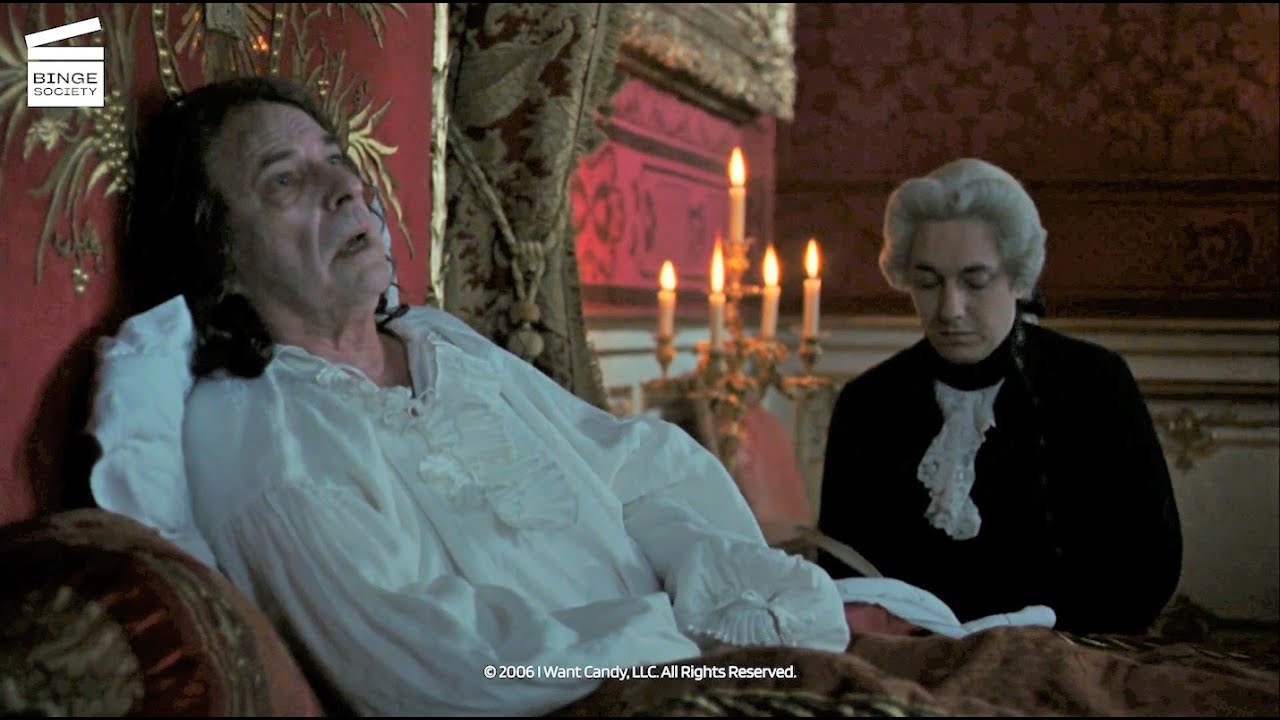The image appears to be a still from a period film or TV show, set in an opulent, palace-like bedroom with red brocade walls and gold detailing. Dominating the foreground is an older, emaciated man who somewhat resembles Alan Rickman but is not immediately recognizable. He has shoulder-length, dark hair, a sickly pallor, and appears deeply despondent or lost in thought, with his mouth slightly open and eyes staring upwards. He is dressed in a luxurious, Victorian-style white silk shirt adorned with ruffles at the wrists and chest. The man is propped up in a lavish bed against ornate, red-and-gold cushions, covered by a subdued brown or salmon-colored blanket.

To his left, seated beside the bed, is another man who appears to be a servant or possibly a clergy member. This man is wearing a black jacket, a high black collar, and a white ruffled cravat. His head is adorned with a coiffed white wig, suggesting a historical setting, perhaps the 1700s or Victorian era. He seems to be reading or writing something, given his downward gaze.

In the background, a candelabra with burning candles casts a warm glow, enhancing the scene's regality. The image is watermarked at the top left with "Binge Society" and a director's clapboard logo, while the bottom displays a copyright notice: "2006 I Want Candy, LLC, All Rights Reserved." The overall aesthetic and details suggest a dramatic, historical narrative, possibly involving themes of royalty, illness, or final moments.